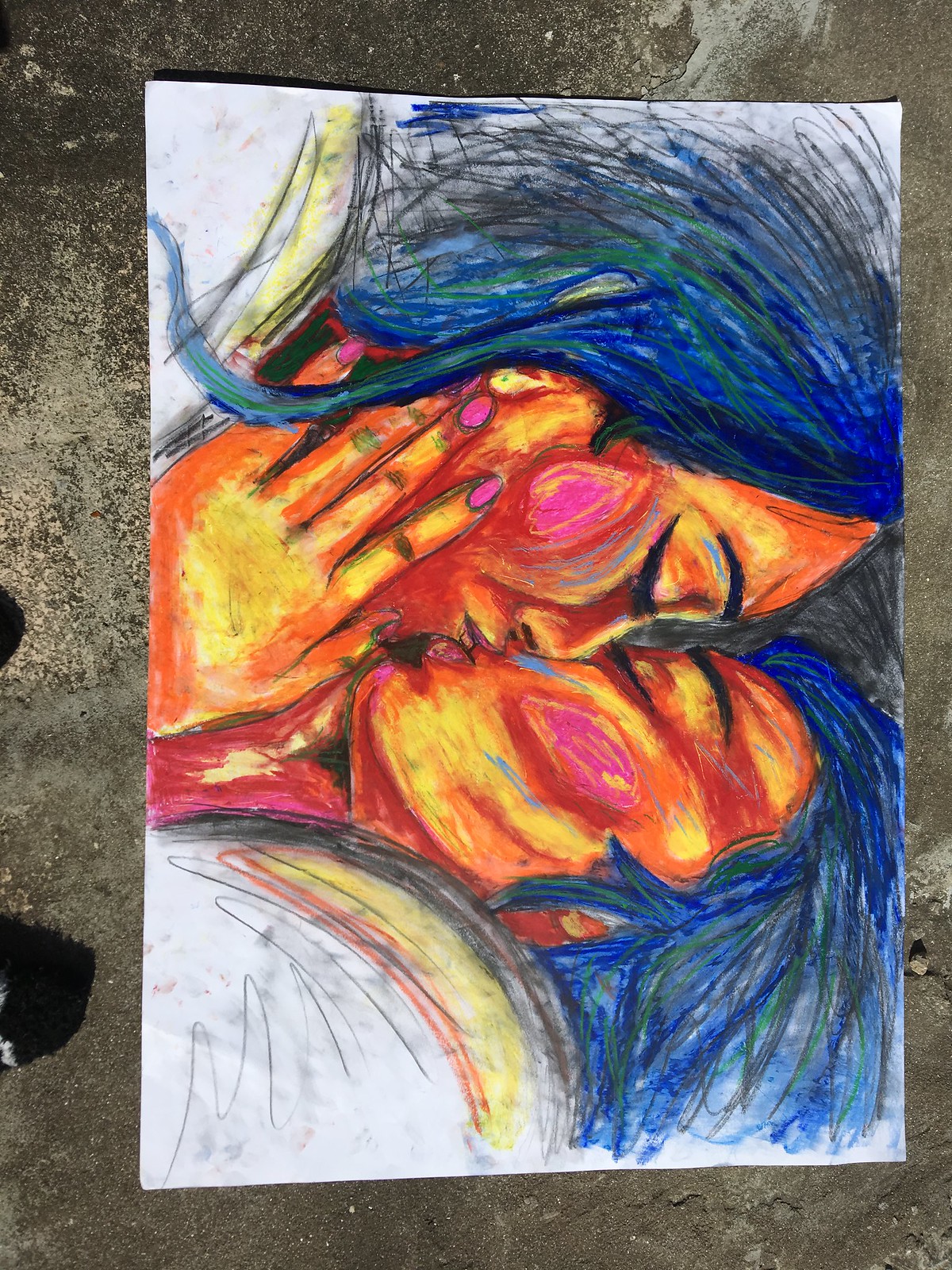This photograph, taken in portrait orientation, features a vividly detailed piece of art lying on a concrete surface. The artwork, likely crafted with oil pastels or colored pencils, depicts two girls engaged in a passionate kiss. Their skin tones blend together in shades of orange, yellow, and pink, with cheeks accentuated by a rosy hue. Both girls have striking hair that mixes blues, greens, and blacks, adding to the dynamic quality of the piece. One girl's hand, adorned with pink nail polish, gently touches the other's face, emphasizing the intimate moment. The artist's use of various colors to create contrast shadows and define details like the black eyebrows and eyelashes, results in a colorful and expressive image. The photo captures the artwork at a 90-degree angle, presenting the couple side-on against a messy, uneven black and grey background, enhancing the raw, emotional impact of the scene.